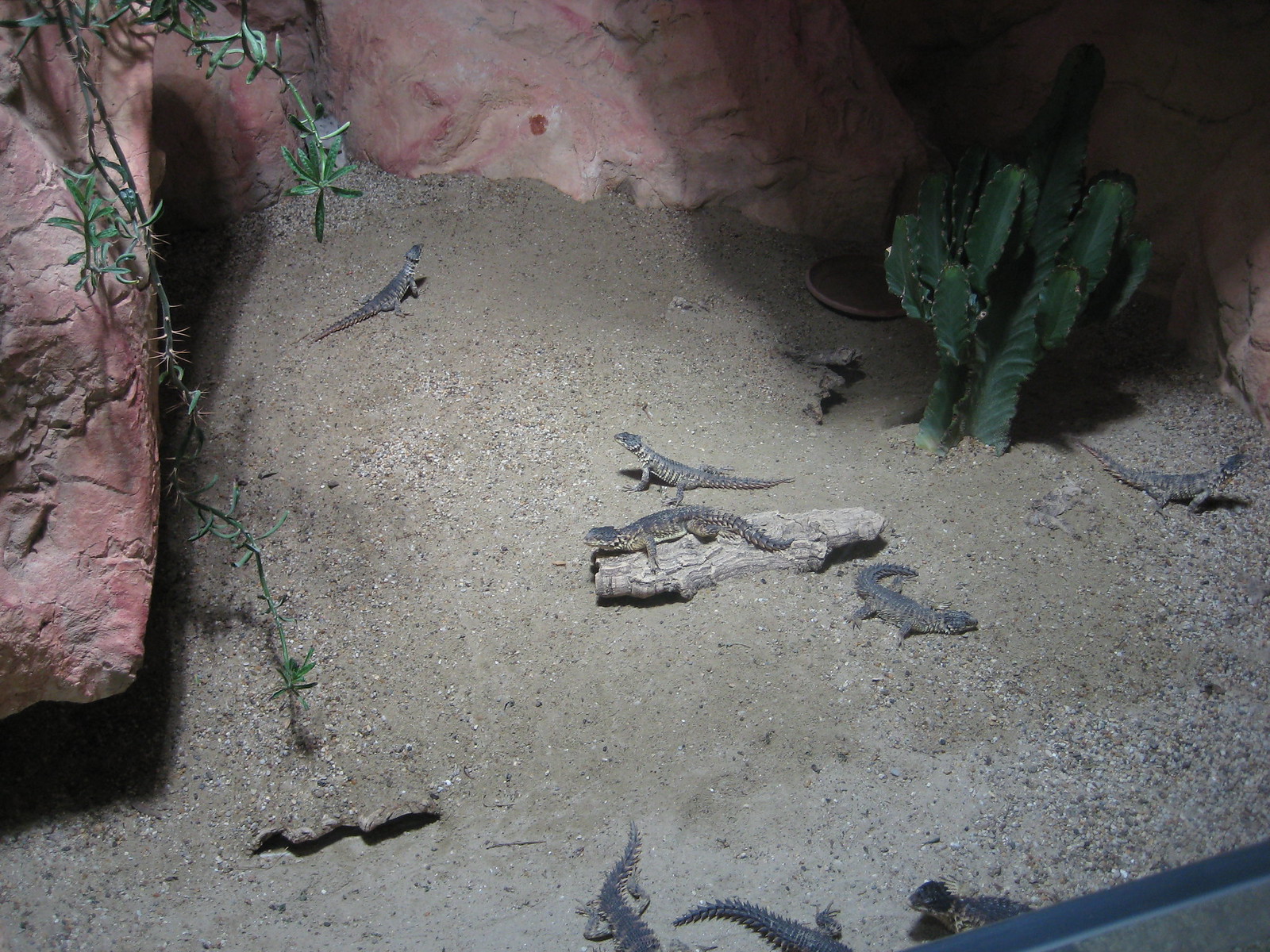The photograph depicts a zoo habitat designed to mimic a desert environment, with a sandy ground featuring grayish-white grains interspersed with small pebbles and rocks. Prominently in the scene, a central piece of dried driftwood hosts a lizard lounging across it, its head oriented towards the left and its tail to the right. The scene includes at least eight small iguana-style lizards, possibly more, blending seamlessly with the backdrop. The habitat showcases reddish, pinkish sandstone-colored rocks, providing a stark contrast to the grainy sand. 

A trailing vine with thorny stems ascends the left side of the image, mingling with the sandstone formation, hinting at a couple of additional lizards camouflaging among the stems. In the dimly lit upper right corner, two small cacti can be seen, alongside what appears to be a food tray, suggesting a managed environment. The top left features a shadowy area, possibly an entrance to a different part of the exhibit. Small plants, including ferns, are scattered throughout, adding to the naturalistic feel of the habitat.